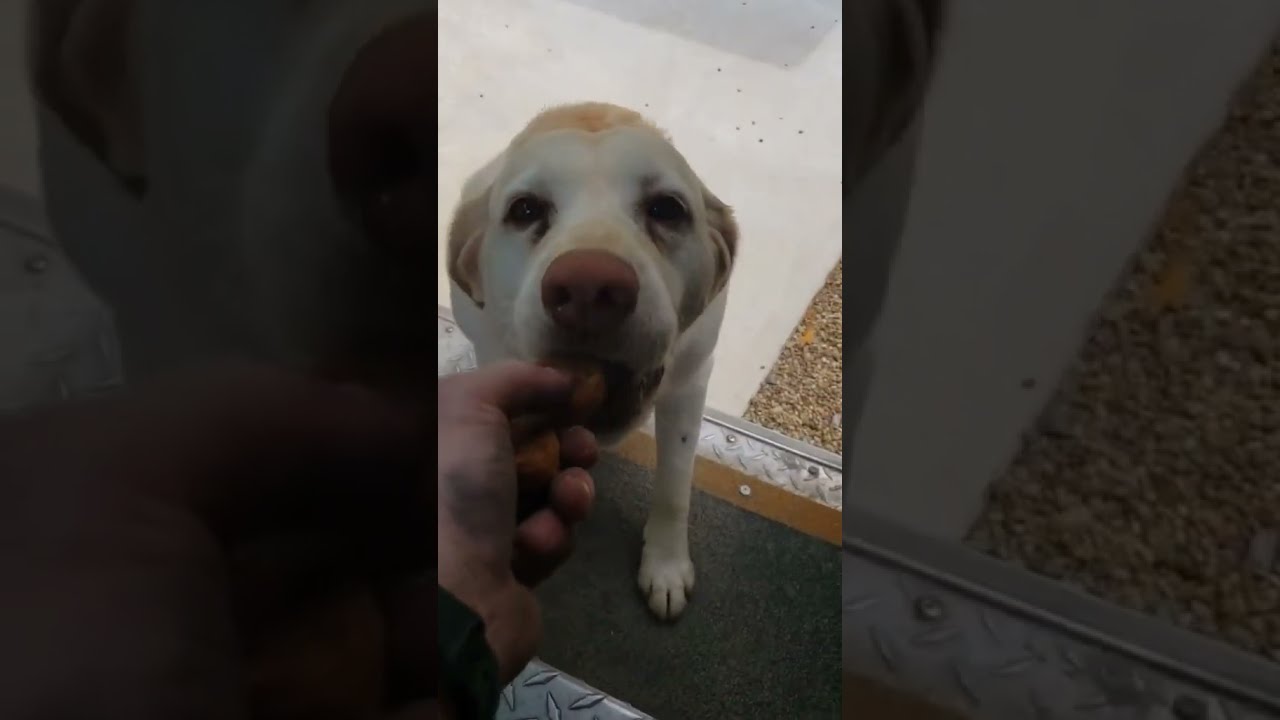In this photograph captured indoors, a large Labrador retriever, prominently white with patches of light brown on its head and brown ears, stands at a doorstep. The dog, featuring a reddish nose and sad, watery eyes, is focused intently on a human hand extending food toward its mouth. The person, partially visible, wears long-sleeved black clothing. The dog’s legs rest on a metallic platform with a black strip in the middle, and the floor behind is white tile. The scene also includes a cement road outside and a patch of brown gravel on the ground to the left. This central image is flanked by two darker, magnified sections highlighting details: the right side focusing on the hand feeding the dog and the dog's nose, while the left side shows the diamond plate and gravel area.